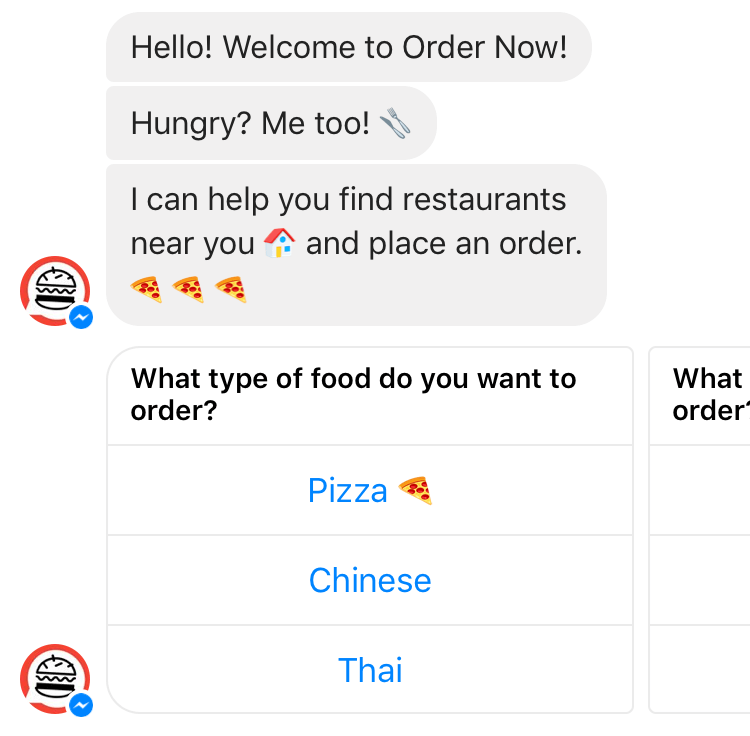The image features a clean white background with several light gray text bubbles containing black text. The first text bubble welcomes the viewer with, "Hello, welcome to Order Now!" followed by, "Hungry? Me too!" accompanied by an emoji of a fork and knife. Below that, another bubble reads, "I can help you find restaurants near you," with a house icon next to it, and "Place an order," with three pepperoni pizza slice emojis.

On the left side, there's a profile picture displaying a segmented circle in red. The circle features a black hamburger illustration in the center and a blue oval with a jagged line. Under this, the text bubble says in bold black text on a white background, "What type of food do you want to order?" Below, two options are presented: "Pizza" with a pepperoni pizza emoji next to it, and "Chinese." To the right, another text bubble prompts, "What's your order?"